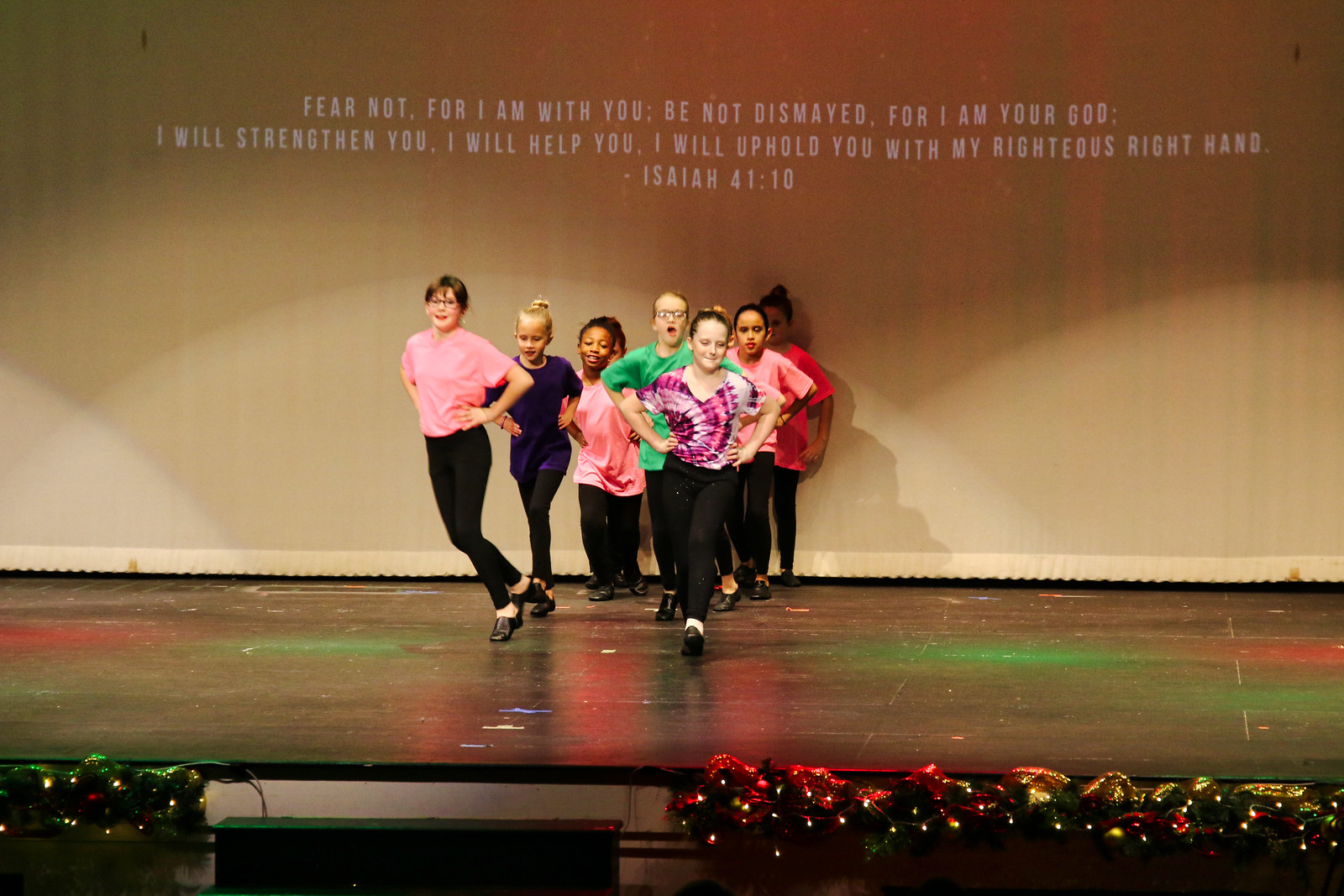The photo captures a lively scene of young girls performing a tap dance on a stage. They are positioned in the middle of the photo, organized into two rows with four girls in each row. All the dancers are wearing black leggings paired with vibrant, colorful short-sleeved tops, including shades of pink, purple, green, tie-dye, and red. Each girl has her hair styled either in a bun or kept very short, contributing to a neat and unified appearance.

The stage is illuminated with various lights, including a spotlight focused on the girls, and features some green and red lighting effects that reflect off the floor. The front of the stage is adorned with little tea lights, adding a charming touch to the setting. Above the girls, the backdrop displays an inspiring message in white text: "FEAR NOT, FOR I AM WITH YOU. BE NOT DISMAYED, FOR I AM YOUR GOD. I WILL STRENGTHEN YOU. I WILL HELP YOU. I WILL UPHOLD YOU WITH MY RIGHTEOUS HAND. ISAIAH 41:10." The girls appear to be enjoying themselves, contributing to an overall joyful and dynamic atmosphere in the photograph.